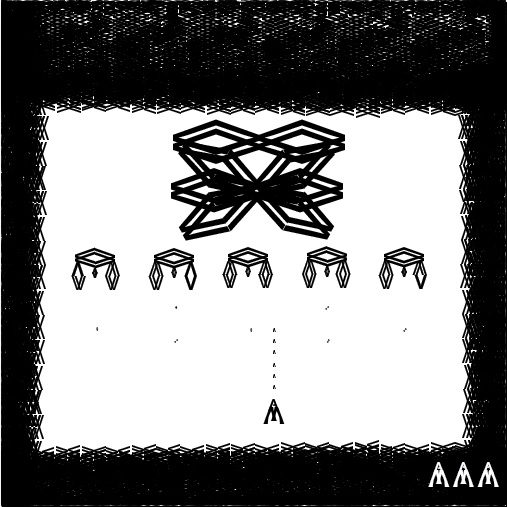This image appears to be a screenshot from a video game featuring a dark maze-like structure set against a high-contrast, monochrome background. The screen is surrounded by a myriad of small, black particles or dots that add to the dynamic visual effect. In the bottom right corner, three white icons resembling upside-down V's with hanging elements can be seen, possibly indicating lives or some form of counter. The main focus of the image is a large, intricate black maze that twists and turns across the screen. Within this maze, five enemy units hover, each shaped like a diamond turned on its side with smaller diamond shapes on either side and a thin protrusion hanging downward. A larger, upside-down V-shaped figure appears to be the player’s avatar or ship, engaged in firing at these hovering enemies, adding an element of action and strategy to the scene.